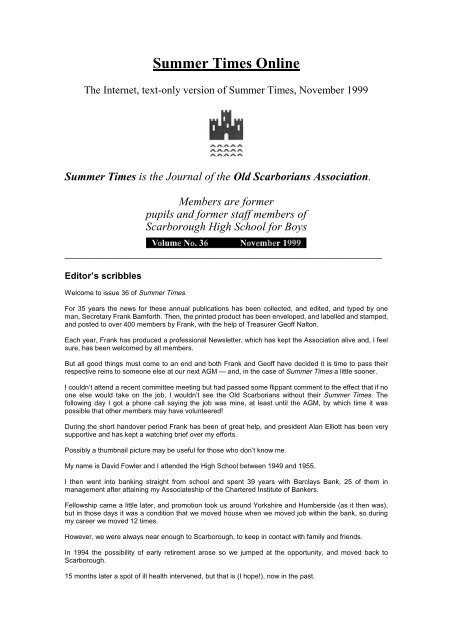In this image, the background is a clean, solid white. At the top, there is a bold headline reading "Summertime's Online," which is underlined in black for emphasis. Below this header, the text identifies the edition as the "Internet text-only version of Summertime's, November 1999." 

A small emblem featuring a stylized castle is prominently displayed, with three rows of small, upside-down V-shaped elements adorning it. The text clarifies that "Summertime's" is the journal of the Old Scarboreans Association, an organization comprising former pupils and staff members of Scarborough High School for Boys. 

There is a distinctive black box containing the publication details: "Volume Number 36, November 1999." Below the box, there are editorial notes, all presented in blueprint style font, introducing the 36th issue of "Summertime's." This section provides a warm welcome to readers and outlines the history and evolution of "Summertime's," paying special tribute to the individual who initiated this annual professional newsletter.